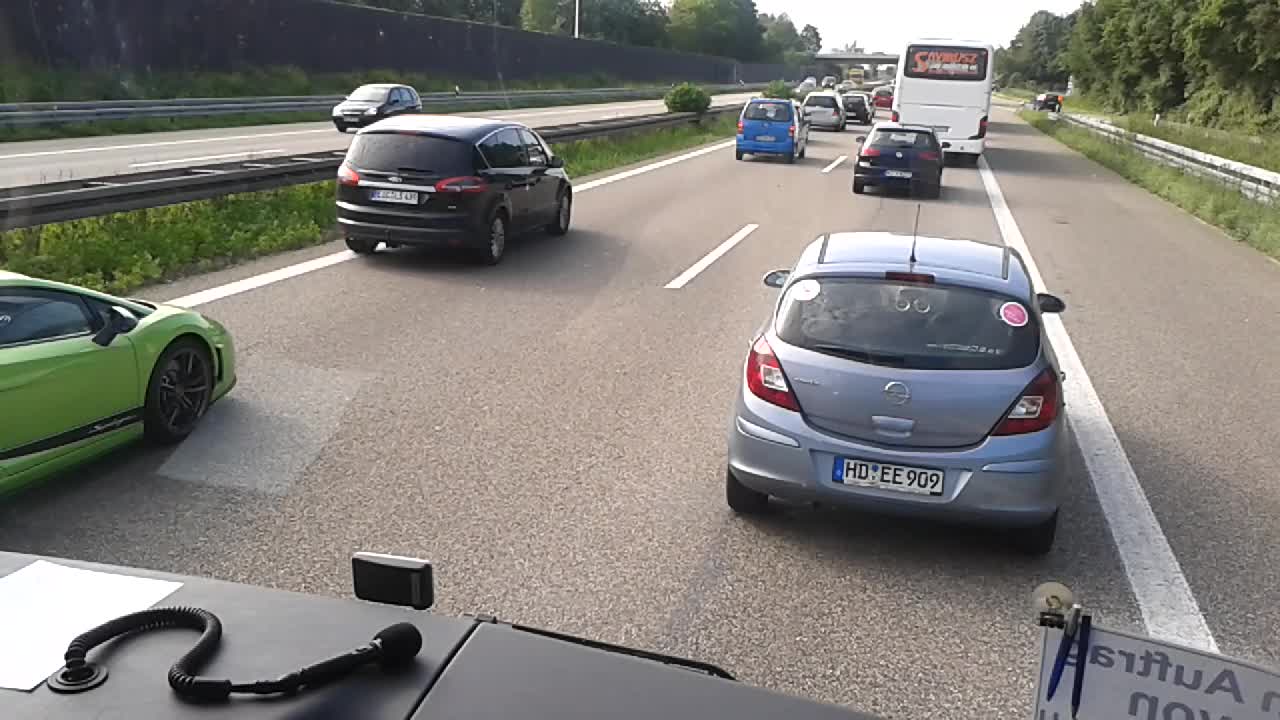The image captures a wider-than-tall, dash cam view from what appears to be a truck traveling down a two-lane highway. The truck's gray dashboard is slightly visible, notably featuring a coiled microphone cord. In the right lane directly ahead, there's a gray car followed by a blue hatchback. To the left, a lime-green car is visible, alongside a black minivan. Further ahead, a white bus with black windows and additional cars are seen progressing down the road. The highway has a dotted white line dividing the lanes, with a shoulder and a guardrail on the right packed with overgrown grass. Trees line both sides of the road, and on the opposite side, separated by a wall, there’s an oncoming black car and other distant vehicles. The setting appears to be outdoors on a clear day, highlighted by the green foliage and orderly traffic flow.